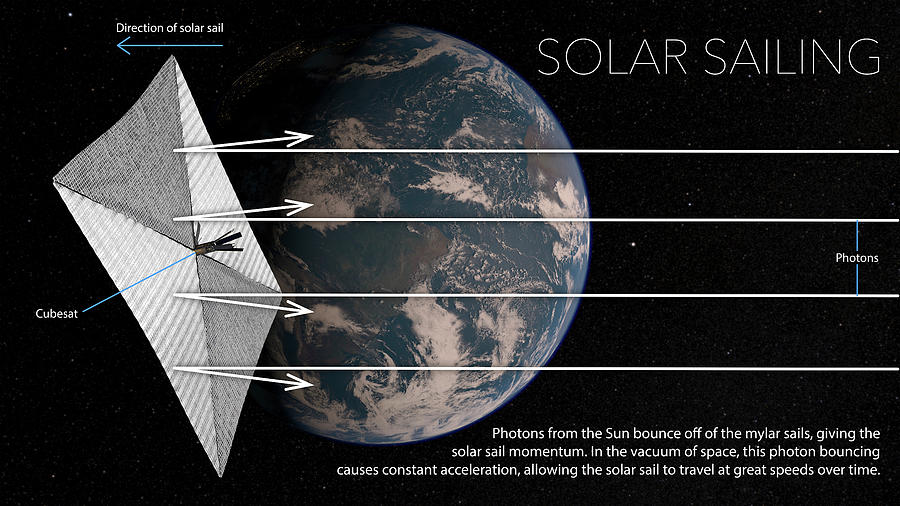The infographic titled "Solar Sailing" illustrates the concept of solar sailing in space. The central focus of the drawing is a diamond-shaped solar sail positioned above the Earth. The Earth is depicted in blue, with white clouds visible against a black background representing space, dotted with stars. 

At the center of the diamond-shaped sail is a labeled "CubeSat," which acts as the sail's core. Four arrows labeled "Photons" approach the sail from the right. Upon striking the sail, these photons reflect and redirect to the left. An arrow above the top of the sail indicates the direction of the solar sail, moving from right to left.

In the bottom right corner, an explanatory caption reads: "Photons from the sun bounce off the Mylar sails, giving the solar sail momentum. The vacuum of space allows this photon bouncing to cause constant acceleration, enabling the solar sail to travel at great speeds over time." 

This detailed visual representation effectively demonstrates how solar sails harness the momentum of photons to propel spacecraft through the cosmos.